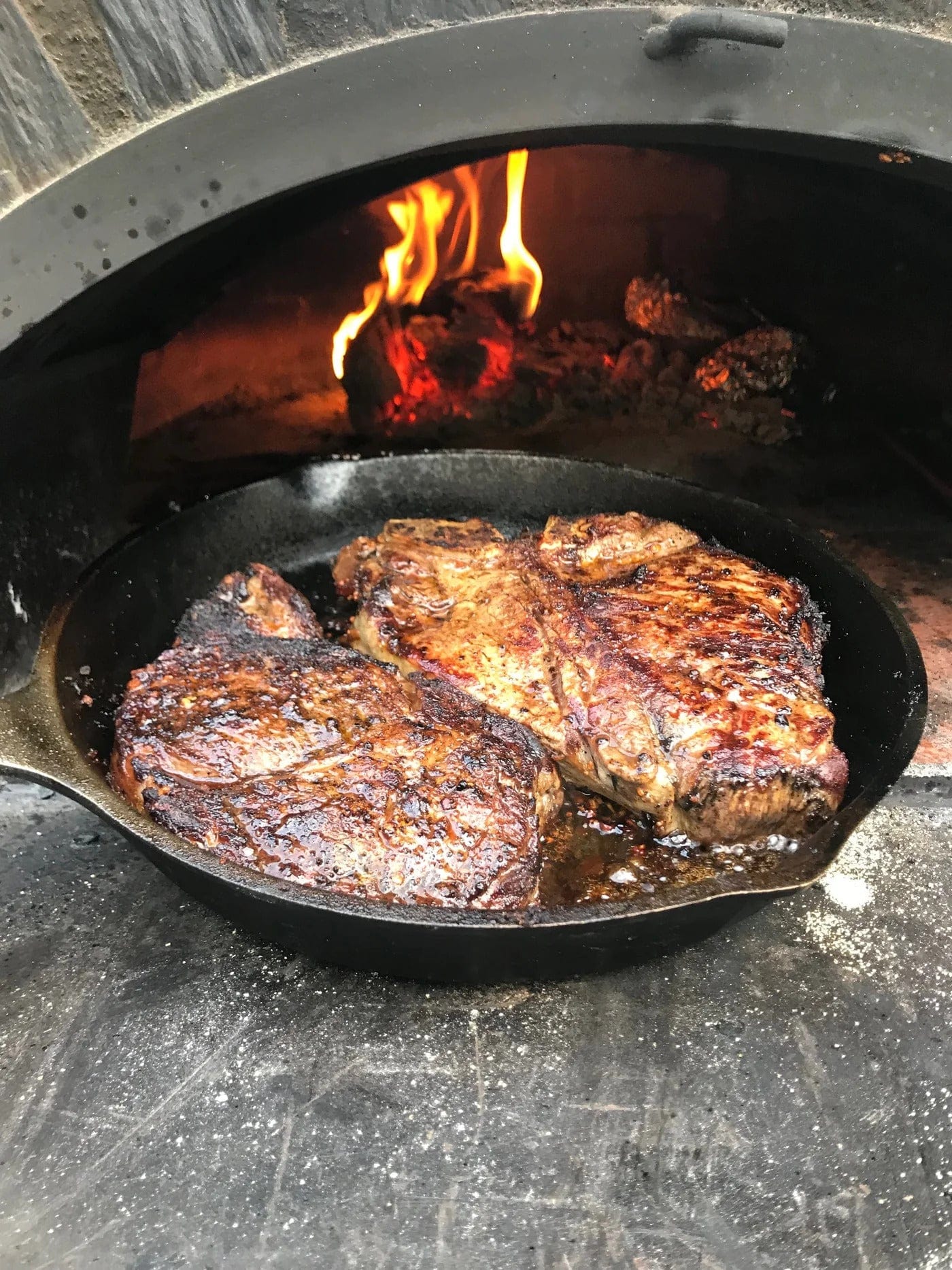The photograph captures a rustic and cozy scene of outdoor cooking. A black cast iron pan, containing two well-cooked beef steaks, rests on a gray metallic or cast iron slab, likely part of a fireplace hearth or an outdoor stove. The steaks are nicely browned and surrounded by rich, dark-colored juices and grease, evidence of a hearty meal in preparation. Behind the skillet, a cast iron arch frames the top portion of the image, leading the eye to a recessed area within the stove where bright red and gray coals burn intensely, emitting vibrant yellow flames. The vertical orientation of the photo gives it a candid, homely feel, reminiscent of something a family member might share on social media, highlighting the simplicity and warmth of cooking by an open fire.